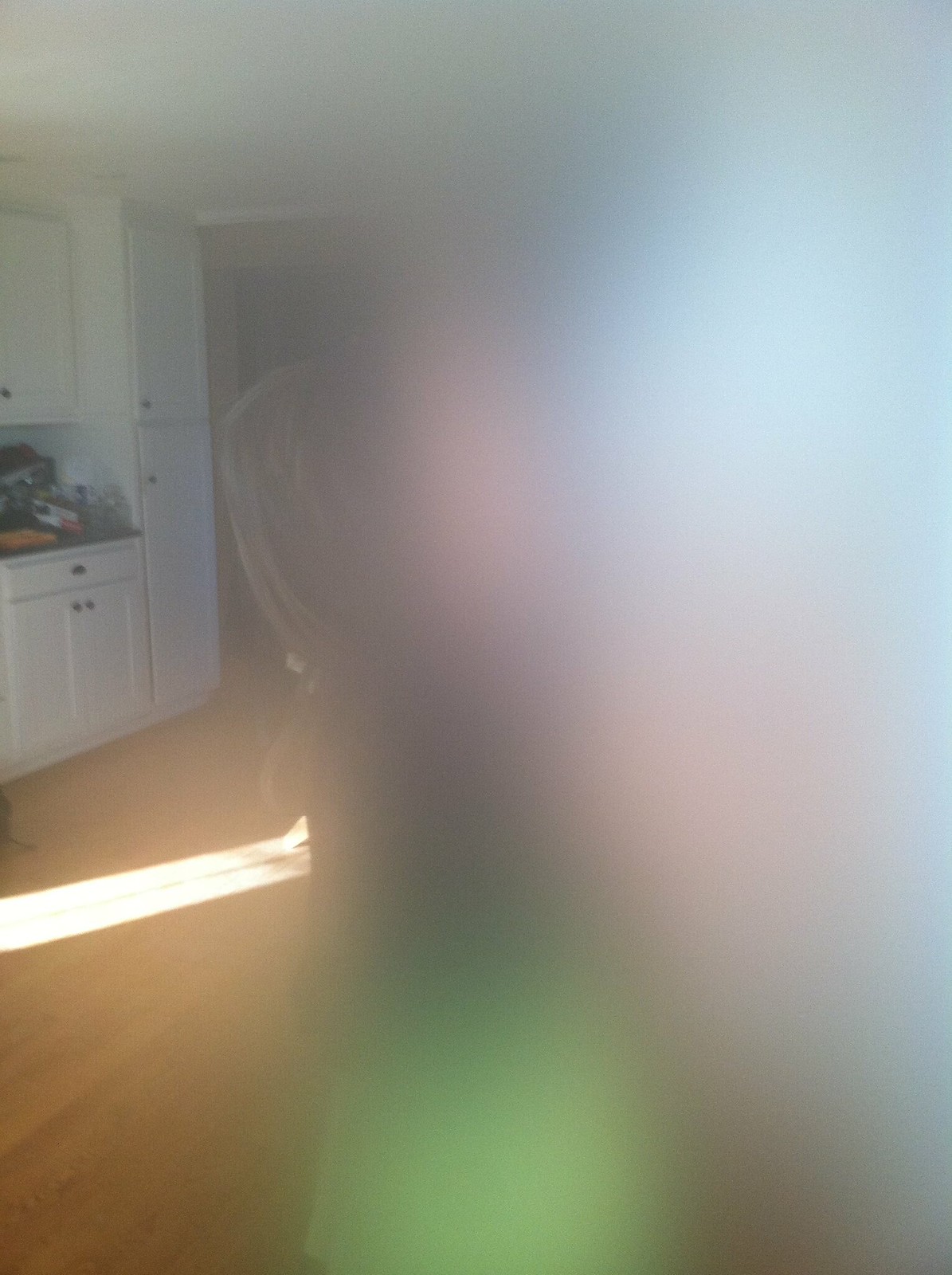This is a color photograph characterized by extreme blurriness, making it difficult to discern specific details clearly. The scene appears to be set inside a home, where the left side of the image offers the most visible elements. Noteworthy is the shaft of sunlight that stretches across a wooden floor, casting a warm, natural light from the top left to the bottom left edge of the frame. Several white cabinets line the left edge of the image, positioned near a cluttered countertop filled with various indistinguishable items. In stark contrast, the right portion of the photograph lacks clarity, presenting only vague white and green shapes that defy identification. It's ambiguous whether this blur results from a photographer’s error or an intentional effort to obscure part of the scene. Overall, the photograph remains an enigmatic representation of a domestic interior, leaving its true details veiled in mystery.